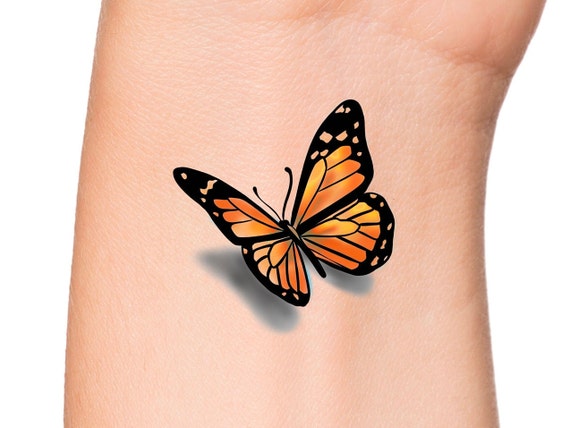The image before us is a digitally created, highly detailed graphic of a monarch butterfly resting on a Caucasian person's wrist. The orientation of the image is such that the shorter side is horizontal. The monarch butterfly features striking black borders around its wings, adorned with white and orange flecks, and inside, the vibrant hues gradient from rich oranges to yellows, with a slight pinkish fade towards the bottom. The butterfly, with its black body and antennae, is positioned facing the upper left corner, casting a dark shadow underneath its wings, suggesting it is a part of the graphic rather than a tattoo. The wrist, which is white with a clear, clean, and pinkish hue, sports visible skin creases on the right side, complementing the crisp quality of the image. The background behind the wrist is a stark white, further emphasizing the intricate details and colors of the butterfly.